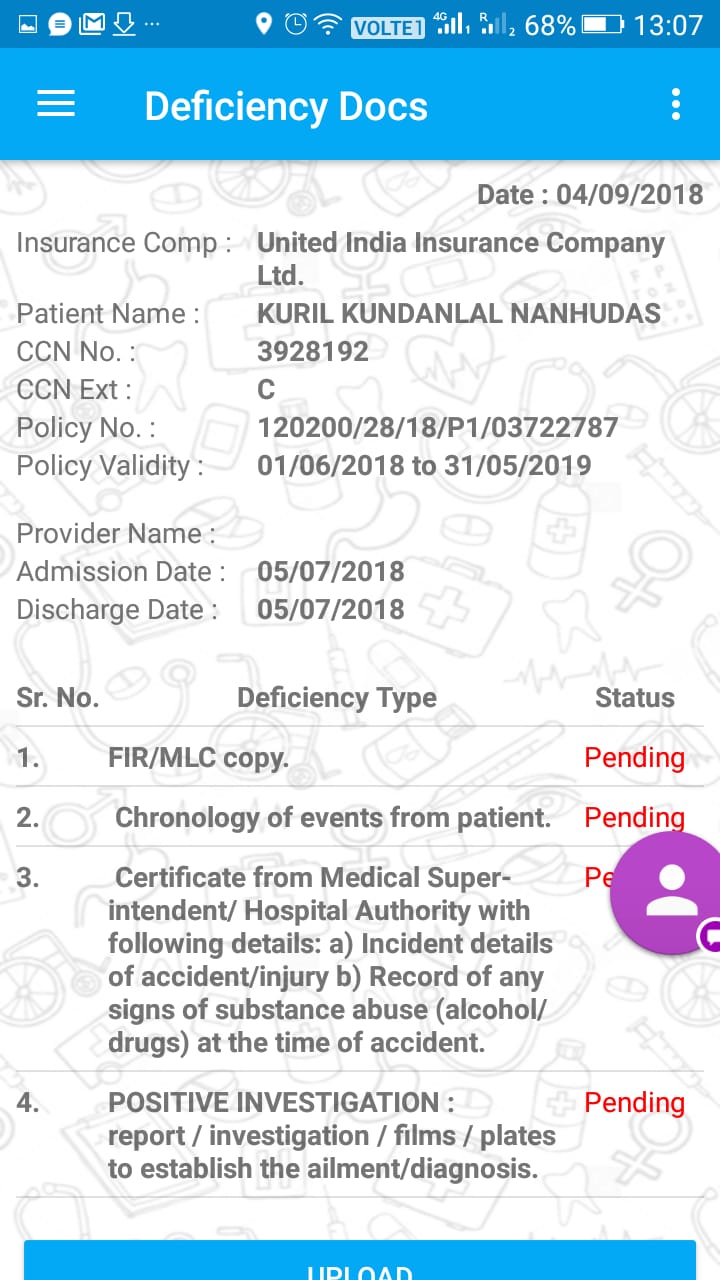This image is a screenshot of a document from an insurance company, indicated by a blue banner across the top with the text "Deficiency Docs" in white font. Dated 04-09-2018, the document is from United India Insurance Company Limited. The patient's name is Kirill Kondulal Nonhudus, with the CCN number 392-28192 and CCN extension C. The policy number is 120200/28/18/P1/03722787, valid from 01-06-2018 to 31-05-2019. The provider's name and the admission and discharge dates are both listed as 05-07-2018. The document details several deficiencies: FIR-MLC copy status pending, chronological events for the patient pending, a certificate from the medical superintendent hospital authority detailing the incident and any substance abuse at the time pending, and a positive investigation report pending. In the background of the document are light gray doodles of medical equipment, and at the top of the screenshot, the phone's status bar indicates a battery level of 68% and the time as 13:07.